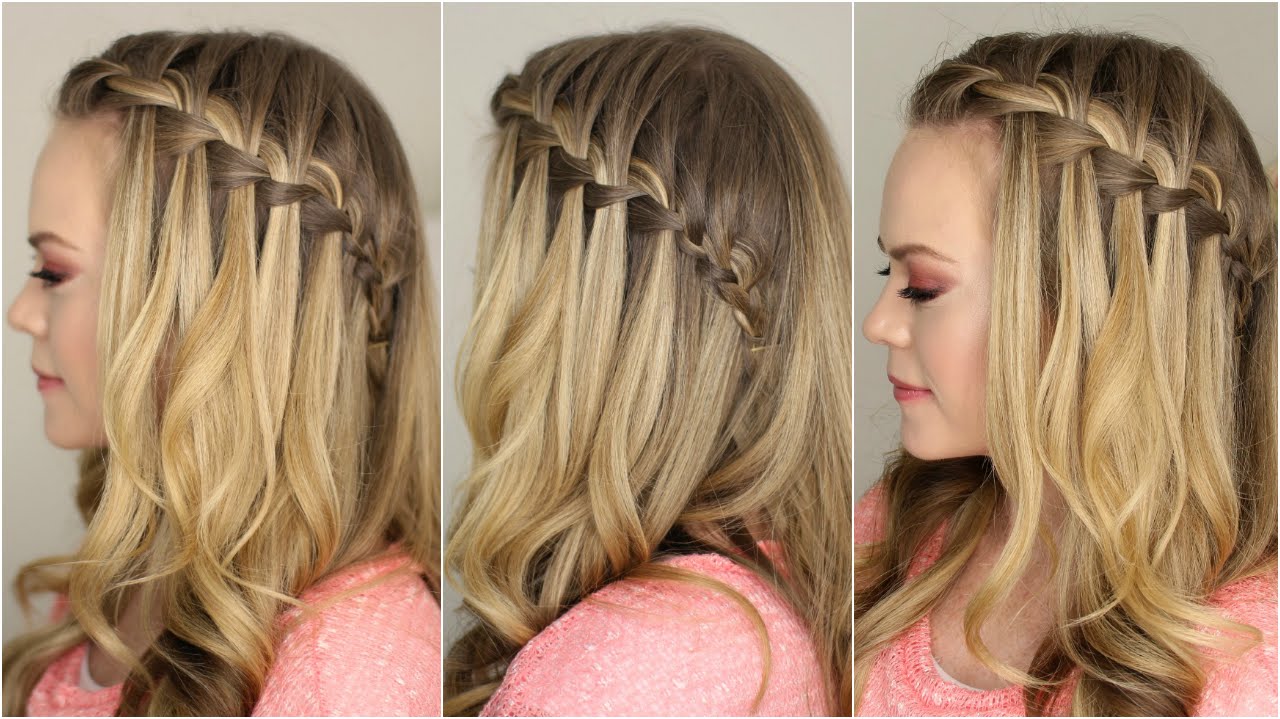This image features three vertically oriented, side-by-side photos of the same young Caucasian woman with fair skin, showcasing different angles of a unique braided hairstyle. The woman has long, lightly curled hair that transitions from brown at the roots to blonde at the ends. A distinguishable front braid starts at the forehead and runs horizontally across her head, merging at the back with the rest of her wavy hair.

She is dressed in a pink shirt with a more muted shade of white or possibly an additional layer underneath. Her eye makeup consists of pink eyeshadow, which complements her pink lipstick and subtle blush, creating a harmonious pastel appearance. The background is a plain gray, ensuring that the focus remains on her and the hairstyle. This detailed series of images likely represents a tutorial from a personal blog, website, or social media account, aiming to guide viewers through the steps of achieving this intricate braided look. 

The photos capture her from different perspectives: the left side view emphasizes the front braid and its integration with her hair; a slightly off-center shot gives a fuller view of her hair and braid; and the right view brings attention back to her facial features and the continuity of the braid. The colors in the image include various shades of pink, red, white, gray, yellow, blonde, and brown, creating a visually appealing and instructional composition.